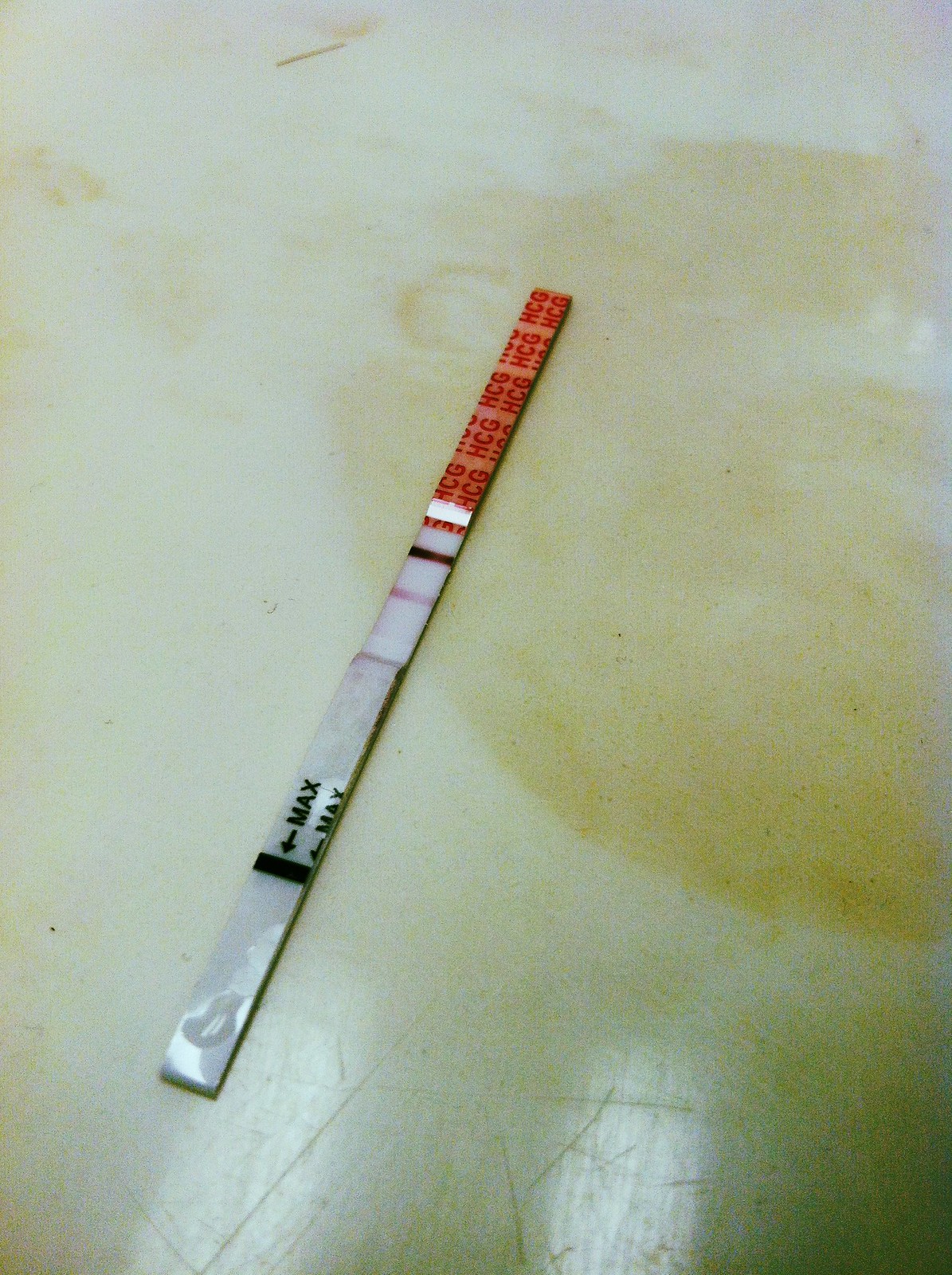The image depicts an old and unsanitary pregnancy test placed on a similarly aged countertop that resembles an old, stained floor. At the top of the test strip, there are multiple segments labeled with "HCG" in red letters. Below these segments, the test features a series of lines in black, red, and white. Near the bottom of the strip, a black line with the word "MAX" and an arrow pointing downwards indicates the required urine level for the test. The test strip itself appears deteriorated, with dark brown discoloration on the top part and a white strip towards the bottom. There is also a drop of liquid—possibly urine or water—visible at the end of the strip. The countertop is white with dark brown stains, giving it an unclean and dated appearance.